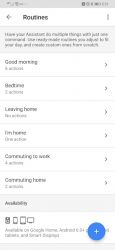**Blurry Mobile Phone Screenshot**

The image is a vertically oriented, blurry screenshot taken from a mobile phone, likely an Android or iPhone. At the top, a gray status bar displays the usual phone symbols such as time (unreadable), battery power, and Wi-Fi, all in a white region. In the top left corner, under the word "Routines" in black letters—blurred but identifiable—there's an indecipherable icon. To the right of this area, a long gray bar with black text includes the words "have your," though the rest are too blurry to discern.

Below this, the interface lists seven interactive options, each separated by faint gray lines. They each feature a clickable gray 'V' on the far right:

1. **Good Morning** (possibly)
2. **Bedtime** with further unreadable text
3. **Leaving Home** with more blurred text
4. Two unreadable options
5. **Commuting to** (likely with unreadable text below)
6. **Connecting House** (possibly with more illegible text below)
7. A gray bar potentially reading **Accessibility**, followed by a white area with a gray rectangle containing a white symbol and three icons that appear to represent computer screens. On the far right of this section, overlapping gray text, is a blue circle with a white plus sign, followed by three gray blocks.

The image quality is notably poor, making further details or text impossible to confirm.